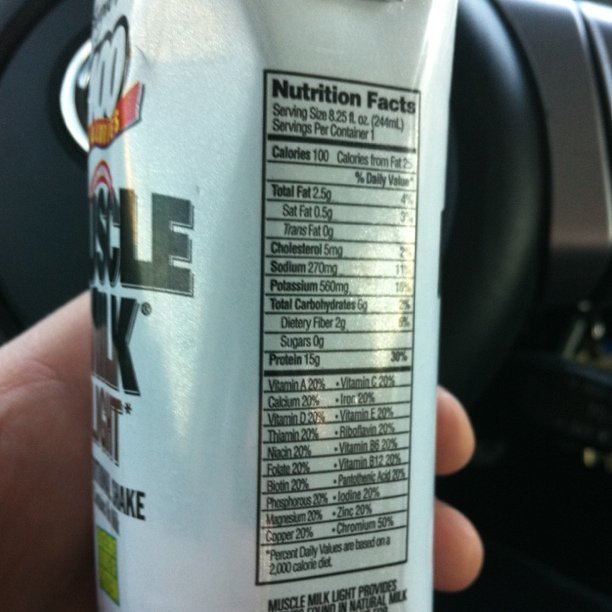The image depicts a carton of Muscle Milk on the left side, where the partially visible text reads "MUSCLE MILK," with letters "S-C-L-E" and "L-K" clearly discernible. The nutritional information is prominently displayed, showing that the serving size is 8.25 fluid ounces, with each serving containing 100 calories. The total fat content is 2.5 grams (4% of the daily value), including 0.5 grams of saturated fat (3% of the daily value), and no trans fat. The detailed breakdown lists cholesterol, sodium, potassium, carbohydrates, dietary fibers, sugars, and proteins, along with vitamins A, C, and E. The text at the bottom mentions something about Muscle Milk Light. In the background, a black steering wheel is visible, and a white man’s hand is holding the carton of milk.